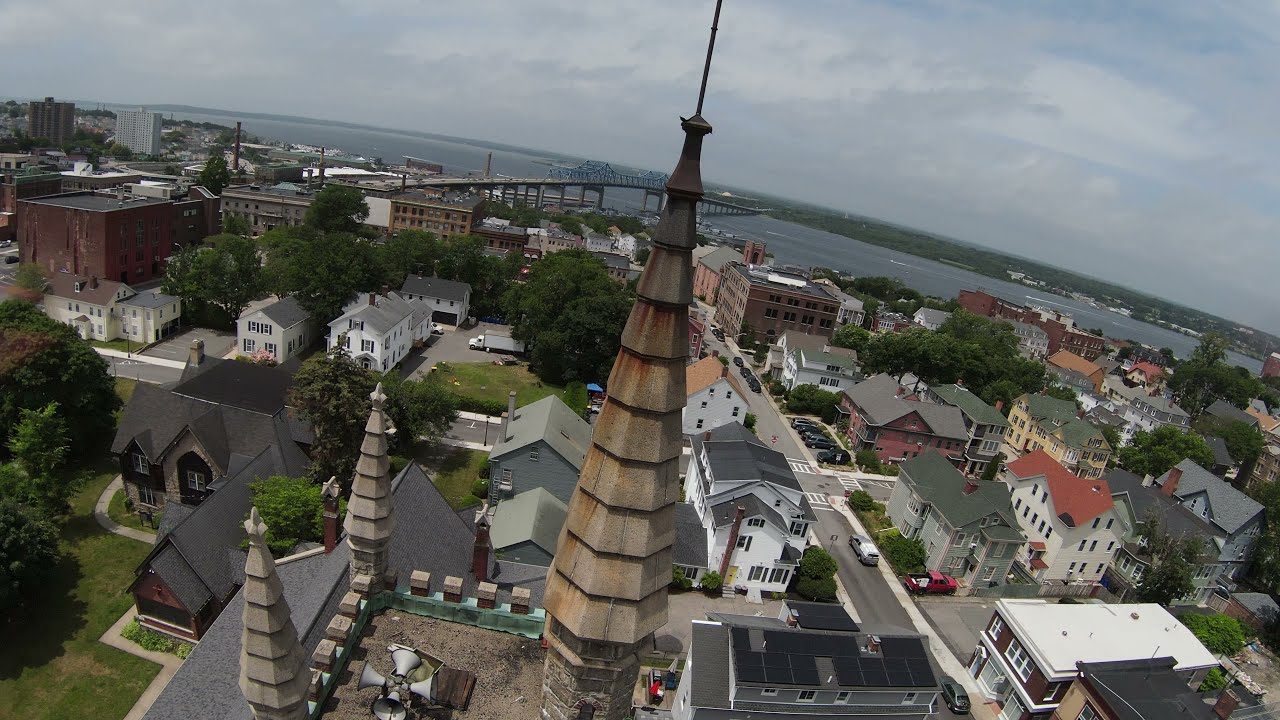The image captures an aerial view of a city during a slightly cloudy day, taken from a drone. Dominating the center of the image is a church steeple, the same height as the drone, topped with a metal rod supporting a cross. Surrounding the church are numerous two to three-story houses painted in varied muted colors—white, gray, and red brick. The neighborhood also features lush green trees and various old-style buildings evocative of a New England town. To the left corner of the picture, a few larger structures are visible, possibly manufacturing buildings or a parking garage. Farther into the background, a stately, expansive bridge spans a river, connecting the city to another landmass. The sky above is filled with light clouds, complementing the serene blue of the water below. The scene is a harmonious blend of architectural elements and natural beauty, captured from an overhead perspective.